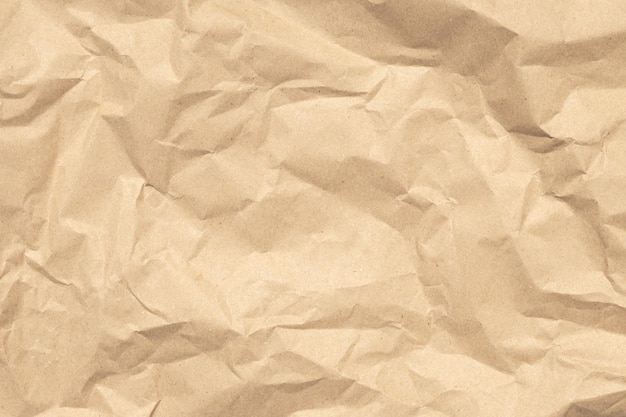This photographic image captures a crumpled piece of light brown or off-white wrapping paper, similar in weight to the kind used for wrapping fragile items in stores. The entire image is dominated by this single crinkled object, with peaks and valleys giving the appearance of miniature landscapes. The upper left quadrant features a pronounced ridge running diagonally towards the bottom right, reminiscent of a mountain range. The middle section shows various blobs and undulating hills, while the bottom left corner has smaller, less pronounced crumples. The top left part of the paper is the most crumpled, with a prominent ridge extending from top left to bottom right. Lighting creates shades of gray within the wrinkles, highlighting the intricate textures and depth of the crinkles, especially in the top right and bottom right corners where the wrinkles are darker and more defined. The paper has been crumpled and then slightly flattened, but retains its complex, crinkled surface with no text or additional elements in the image.